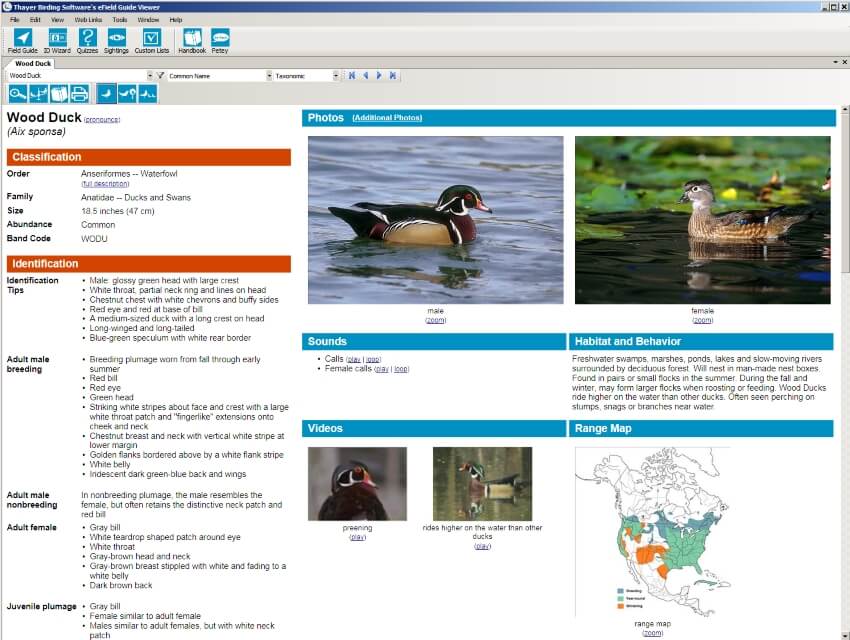This screenshot captures a vintage web page dedicated to the Wood Duck, featuring a layout reminiscent of older web browsers. Prominently at the top is a narrow gradient blue bar, darkening from right to left. Below this bar, two rows of light blue squares with different options are aligned horizontally, lending a dated yet systematic feel to the design.

Below these rows, the black text "Wood Duck" is centrally displayed. The left section of the page features an orange background with two main headers: "Classification" and "Identification," followed by detailed notes occupying the bottom half.

On the right side, a blue background banner labeled "Photos" in white text showcases side-by-side images of two Wood Ducks. The left photo shows a duck swimming in clear water, while the right displays a duck in almost black water with lily pads in the background. Each bird is depicted in a side profile, allowing for easy comparison. Beneath the photos, the labels "Male" on the left and "Female" on the right help in distinguishing the sexes of the ducks.

Further down, a section titled "Sounds" is followed by another labeled "Habitat Behavior," accompanied by a descriptive paragraph. The bottom left area features a section for videos, while the right side concludes with a "Range Map," displaying an animated map with regions highlighted in orange, turquoise, and light blue.